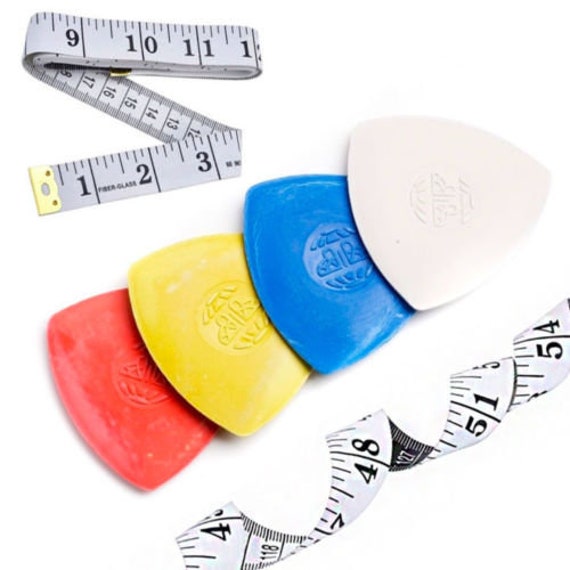The photograph captures a minimalistic and professional image of four colorful guitar picks—red, yellow, blue, and white—arranged centrally on a pristine white background. Each pick, which shows signs of wear with visible scratches, features a faint circular stamp in the center, likely representing the brand logo. Surrounding the guitar picks are two flexible measuring tapes: the one on the top left is a thin gray tape shaped into a horizontally flipped "C," while the one at the bottom right is a black-and-white tape curled into a spiral. The careful arrangement and high-quality lighting emphasize the simplicity and details of the objects, creating a balanced and visually appealing composition.